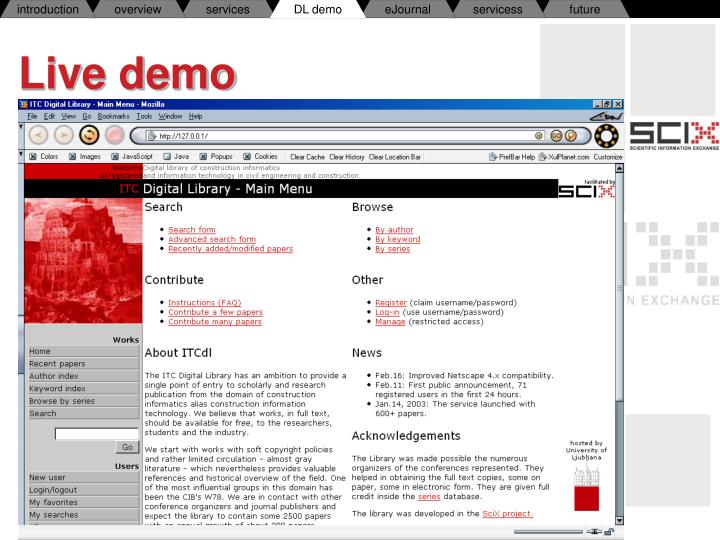The image is a detailed, dated screenshot of a computer window, likely from an older operating system such as Windows 98 or XP. The focal point of the image features a browser displaying a digital library interface. At the very top of the window are various tabs labeled: Introduction, Overview, Services, DL Demo, E-Journal, Services, and Future. The upper left corner boldly shows 'Live Demo' in red text. There's a classic window styled with 90s aesthetics, including a website link and sections labeled Digital Library, Main Menu, Search, Contribute, About, ITC DL, News, Other, Browse, and Acknowledgements. On the left side, a gray sidebar shows options including Home, Recent Papers, Author Index, Keyword Index, Browse By Series, Search Box, New User, Log In, Log Out, My Favorites, and My Searches. The visual palette consists mainly of gray, black, white, and red colors, adorned with the SCIX logo on the right side of the window. The entire scene gives off a nostalgic vibe of early internet browsing, suggesting an academic or research-oriented setting. The background includes rocky red mountains to the left, indicating a blend of digital and geographic elements.